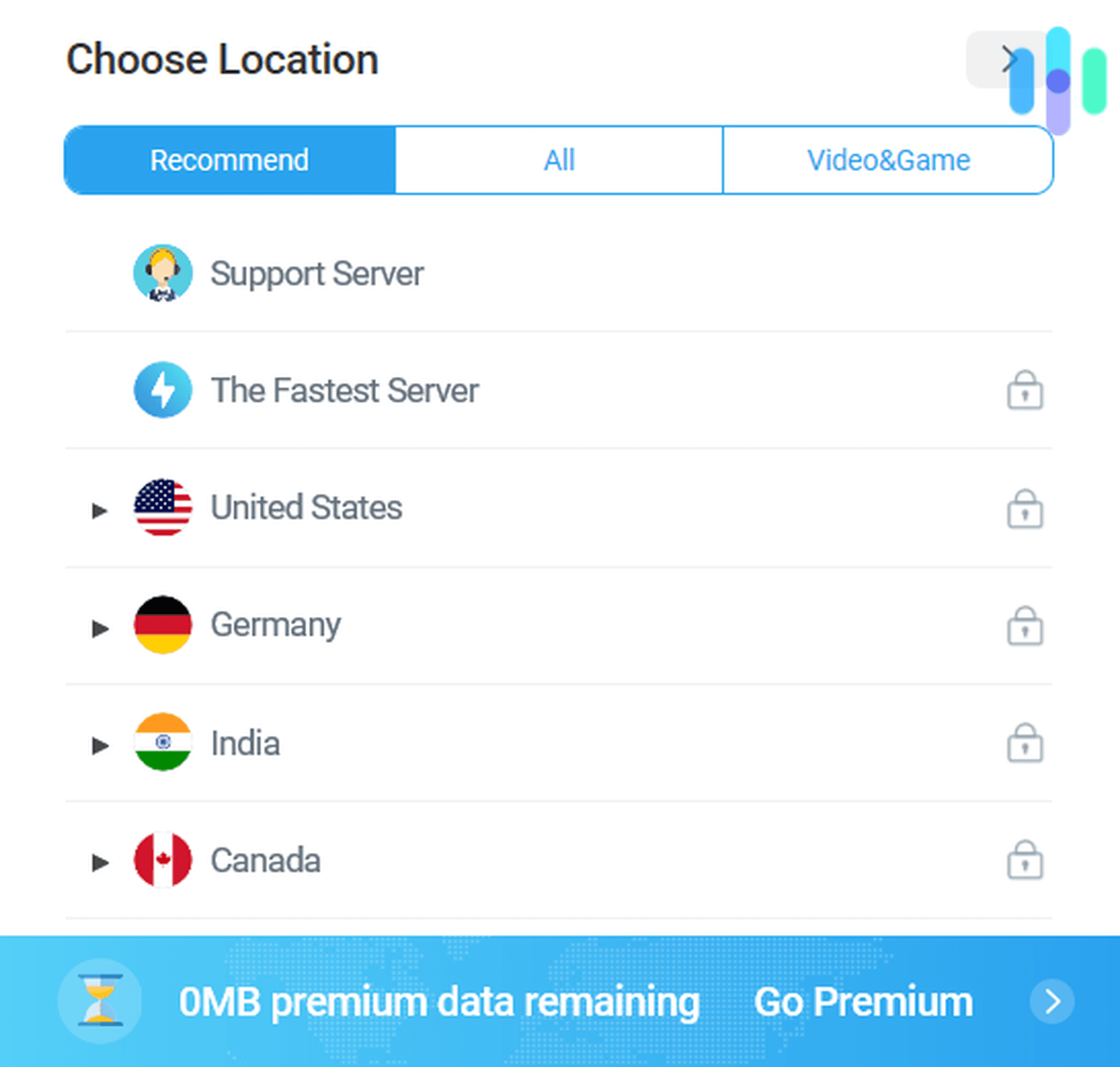The image shows a screen with a user interface for selecting a location. At the top, the title "Choose Location" is displayed in black text, accompanied by an icon featuring colorful lines—one in blue, another in a lighter blue transitioning to purple, and a third in green.

Beneath the title, there are several tabs organized into categories: "Recommended," "All," "Video," and "Game." These tabs are highlighted in blue, with the "Recommended" tab in a darker shade of blue, indicating it is the currently selected page.

The screen lists different connection options, each with distinct icons. The "Support Server" has an icon of a customer support person, and the "Fastest Server," marked by a lightning bolt icon, is accompanied by a lock icon signifying it is secured.

Various country options are presented, each showing its national flag and a lock icon, denoting restricted access. 
- The United States is represented with the red, white, and blue flag.
- Germany features its black, red, and yellow flag.
- India shows the orange, white, and green flag.
- Canada is depicted with the red and white flag.

At the bottom of the screen, an hourglass icon indicates "0 MB premium data remaining," and nearby, a "Go Premium" button with a right-pointing arrow on a blue background encourages users to upgrade. The majority of the page features black text on a white background, ensuring clear readability.